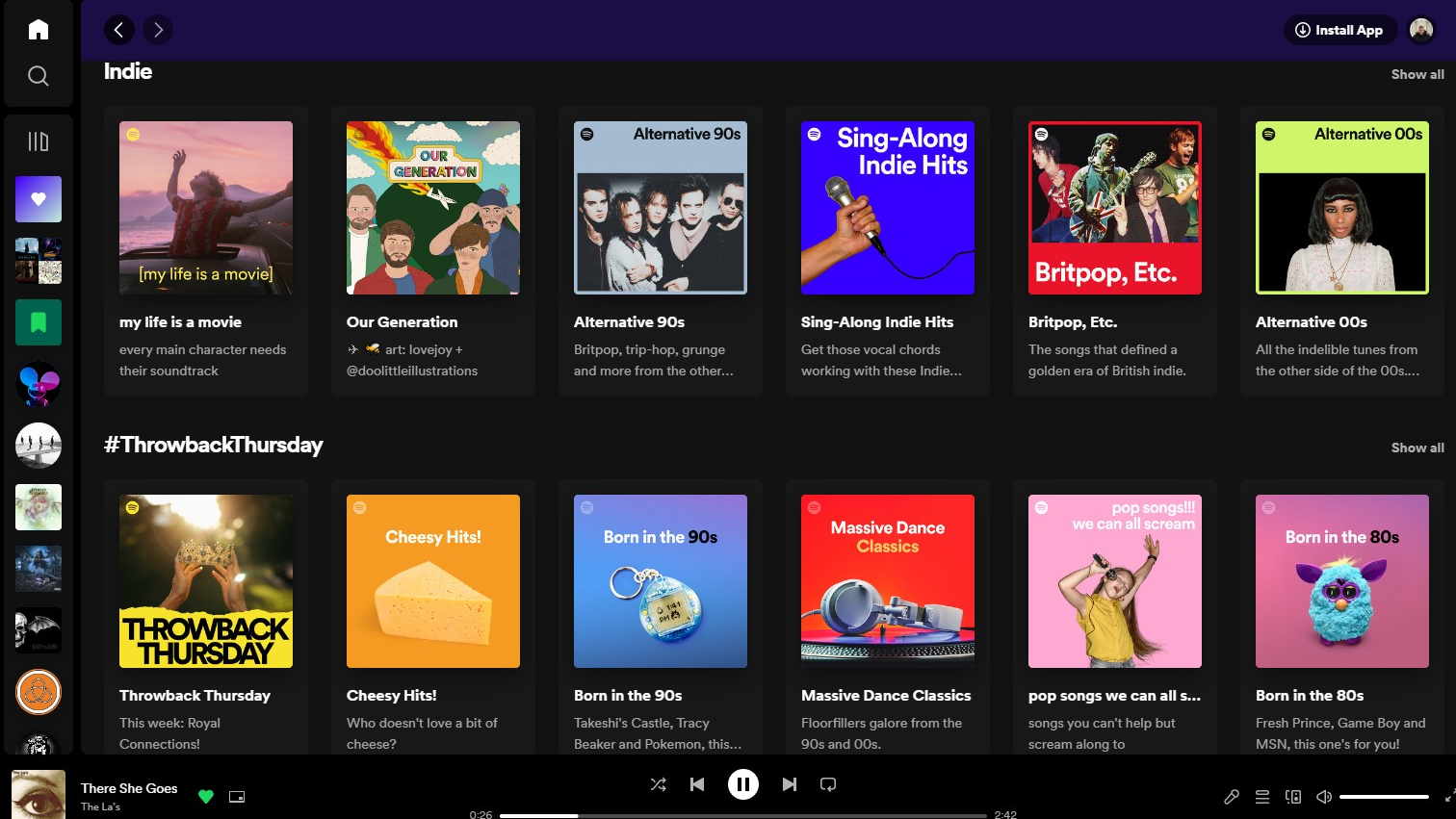This is a screenshot from an unidentified music-based application, featuring a dark-themed interface. At the top section, we see the category "Indie" alongside options to "Install App" and "Show All." The highlighted text reads: "My life is a movie. Every main character needs their soundtrack. Our generation: art, love, joy, little illustrations." Below these words, various music categories and playlists are showcased:

- **Alternative 90s**: Explore Britpop, trip-hop, grunge and more from this transformative era.
- **Sing Along Indie Hits**: Engage your vocal cords with these indie anthems.
- **Britpop, Etc.**: Timeless songs that encapsulate the golden era of British indie music.
- **Alternative 00s**: Unforgettable tracks from early 2000s alternative scenes.
- **Throwback Thursday**: Celebrating Royal Connections this week.
- **Cheesy Hits**: Guilty pleasures you can't resist.
- **Born in the 90s**: Nostalgic titles like Takeshi's Castle, Tracy Beaker, and Pokémon.
- **Massive Dance Classics**: Floor fillers from the 90s and 00s sure to get you moving.
- **Pop Songs We Can All Scream**: Irresistible anthems to belt out.
- **Born in the 80s**: A tribute to the iconic era featuring Fresh Prince, Game Boy, and MSN.

In the bottom left corner, the current track playing is "There She Goes" by The La's, accompanied by album artwork showcasing a dramatic closeup of a woman’s left eye accentuated with heavy eye makeup.